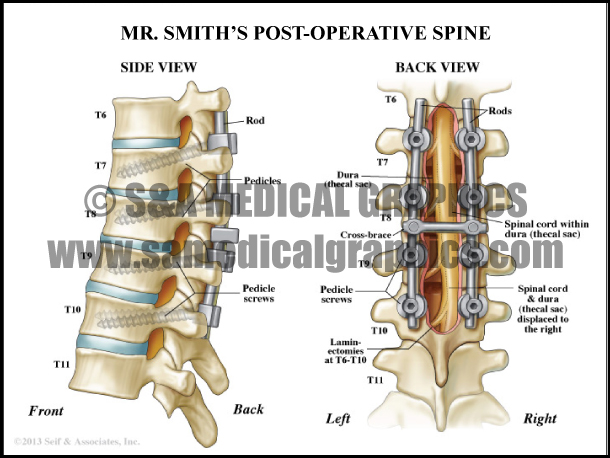The square image features a black border on a white background, prominently titled at the top in black, all-caps letters: "MR. SMITH'S POST-OPERATIVE SPINE." Below the title, the image is split into two labeled sections: "SIDE VIEW" on the left and "BACK VIEW" on the right. 

The "SIDE VIEW" section illustrates the spine from a lateral angle, highlighting vertebrae T6 through T11. A metal rod runs through the vertebrae, with labels such as "Rod," "Pedicle Screws," and directional markers "Front" and "Back." Arrows point to various labeled parts including "Pedicles" and "Cross Brace."

The "BACK VIEW" section shows a posterior angle of the spine with two rods alongside the spinal column. Key annotations include "Spinal Cord within Dura," "Spinal Cord and Dura," "Dura," "Pedicle Screws," and "Laminectomies at T6 and T10." Verbal markers indicate "Left" and "Right" sides of the spine.

Translucently printed across the center of the image in a grey block font is a copyright mark indicating "SNA Medical Graphics," along with a partially obscured website, "www.SNAMEDICALGRAPHICS.com."